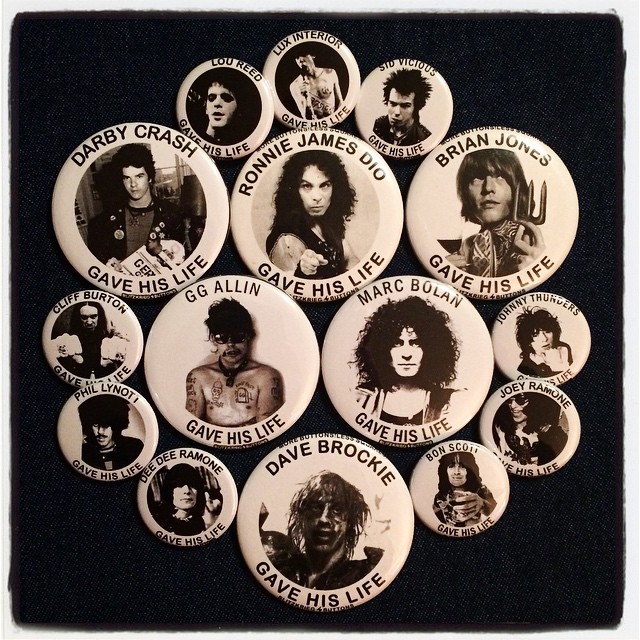The image is a large square with a solid black fabric background, evidenced by small fuzzes and imperfectly smooth edges. On this background, there is a detailed arrangement of black-and-white pins featuring rock stars who each "gave his life." The pins form an inverted pyramid with three large ones at the top, followed by two more in the middle row, and a single one at the bottom. Notable larger pins include Darby Crash, Ronnie James Dio, and Brian Jones from the top down, and Gigi Allen and Mark Bolan in the bottom row. Surrounding this main pyramid are smaller pins, nine in total, positioned to the left, right, and above, creating a circular pattern. These smaller pins represent figures like Sid Vicious, Lux Interior, Lou Reed, Cliff Burton, Johnny Thunders, Joey Ramone, Dee Dee Ramone, Don Scott, and Phil Lynott. Each pin displays a photo of the musician with their name and the phrase "gave his life" inscribed at the bottom, capturing the essence of rock legends from the 60s to the 80s.